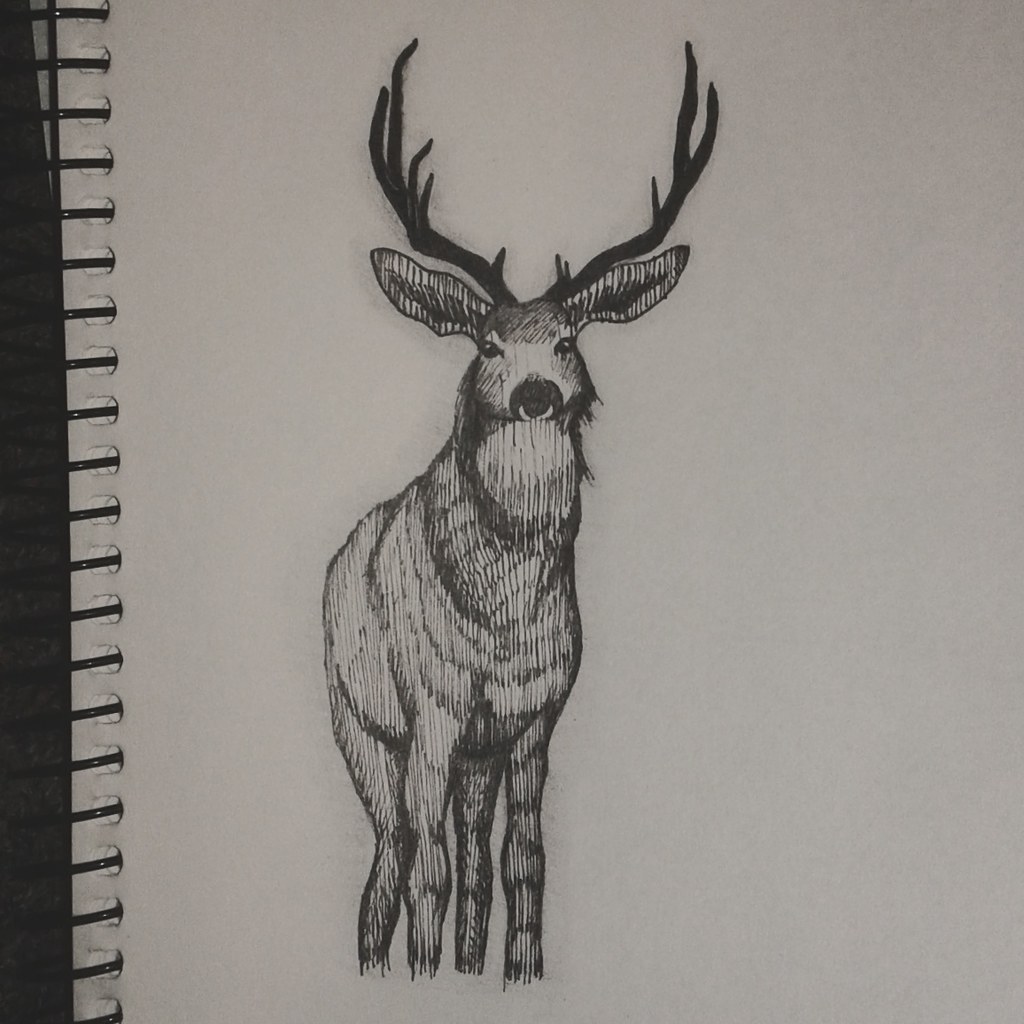In this detailed black-and-white pen and ink drawing on a white sheet of paper from a spiral-bound sketchbook, a majestic and imposing male deer stands tall, gazing directly at the viewer. The paper's black spine is visible on the left side, showcasing the characteristic holes of the sketchbook. The deer, meticulously illustrated, features enormous tree-branch-like antlers, long ears, and a prominent black nose that almost appears to have a ring. Its eyes, with sharply defined black and white pupils, add to its lifelike appearance. The body of the deer is covered in intricate linework to simulate thick fur, which extends down all four visible legs, though the hooves and tail are not depicted. The stance of the deer, head held high and eyes fixed forward, combined with its well-detailed fur and shading, gives it a somewhat intimidating yet realistic presence at the center of the composition.